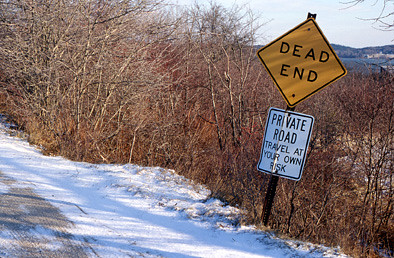In the photograph, a yellow diamond-shaped "Dead End" sign with black lettering prominently stands on the left-hand side of the snow-covered road. Below it, a white rectangular "Private Road, Travel at Your Own Risk" sign with black lettering is attached, both slightly leaning to the right. The road itself, located diagonally to the left, has been scraped clear of snow, though a couple of feet of snow remain piled higher on the sides.

Surrounding the road, the landscape features an abundance of brown, leafless trees and bushes, interspersed with patches of red, dead leaves. In the distant background, a range of mountains is faintly visible beneath the overcast, white sky. It's likely midday or early afternoon, as indicated by the soft shadows cast on the snowy ground.